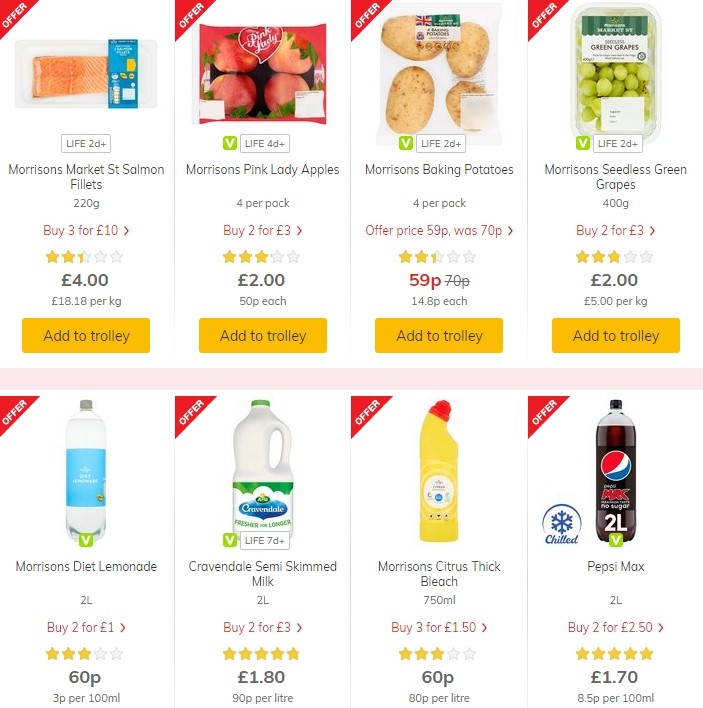The screenshot captures the desktop view of the Morrisons' website, a UK-based grocery store offering online shopping and home delivery services. Prominently displayed are various grocery items currently on special offer. The highlighted products include a salmon fillet, Pink Lady apples, baking potatoes, seedless green grapes, Morrisons Diet Lemonade, Cravendale Semi Skimmed Milk, Morrisons Citrus Thick Bleach, and Pepsi Max, with the latter notably priced at £1.70 or two for £2.50. Interestingly, except for the Pepsi Max and the Semi Skimmed Milk, most items have received ratings of three stars or below.